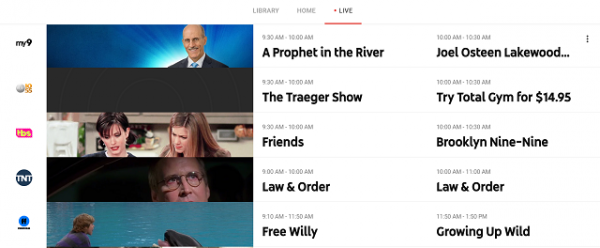The image is a white rectangle featuring a photo collage on the left side. Running vertically next to the collage, there are five distinct icons whose details are partially discernible, including the labels for "TBS" and "TNT." 

At the top of the collage, there is a photograph of a man against a navy blue background. He is dressed in a black suit with a white shirt and a tie. Only his head and shoulders are visible; he has a mustache and is bald.

Below this, there is a black rectangle with no visible content. Further down, there is another rectangle featuring two women from the TV show "Friends" — a younger Jennifer Aniston and Courteney Cox. 

Underneath, there is an icon with a black background that includes an image of a man wearing glasses with "Law and Order" written to the right side of it. Below this, there is an image from the movie "Free Willy," showing the young boy and the whale, only partially visible.

To the right of the image collage, text proceeds from top to bottom, organized into two columns. The first column reads: "A Prophet in the River," "The Traeger Show," "Friends," "Law and Order," and "Free Willy." The second column includes: "Joel Osteen Lakewood," "Try Total Gym for $14.95," "Brooklyn Nine-Nine," "Law and Order," and "Growing Up Wild."